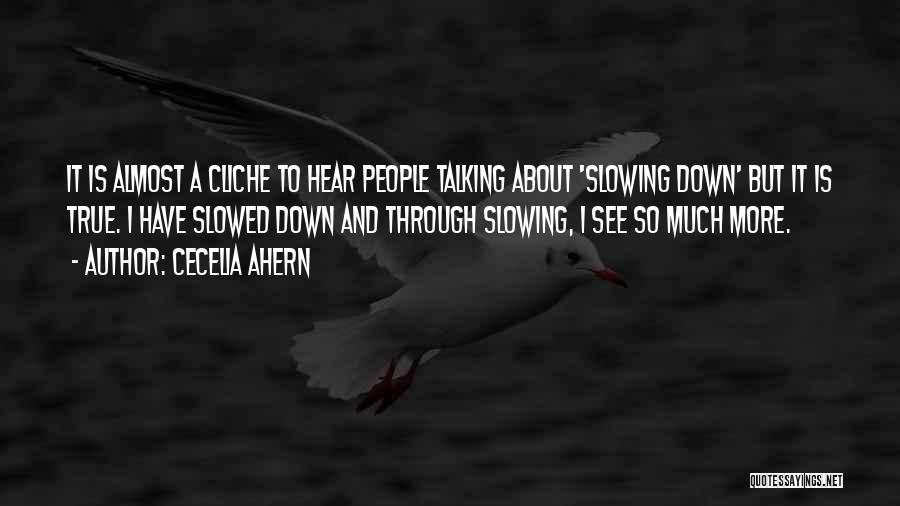The image is mostly dark, with a black and gray color palette accented by hints of orange and red. A light-colored bird, possibly a dove or seagull, is centered in the picture, flying over the water with its wings spread wide. The bird has a distinctive orange-red beak and black spots around its eyes. Across the center of the image, overlaid on the bird, is a quote in white font from author Cecilia Ahern: "It is almost a cliché to hear people talking about slowing down, but it is true. I have slowed down and through slowing I see much more." In the lower right corner, a small white box contains the text "Quotesayings.net" in black letters. This image, with its profound message and centered composition, has the aesthetic of something that might be shared widely on social media.